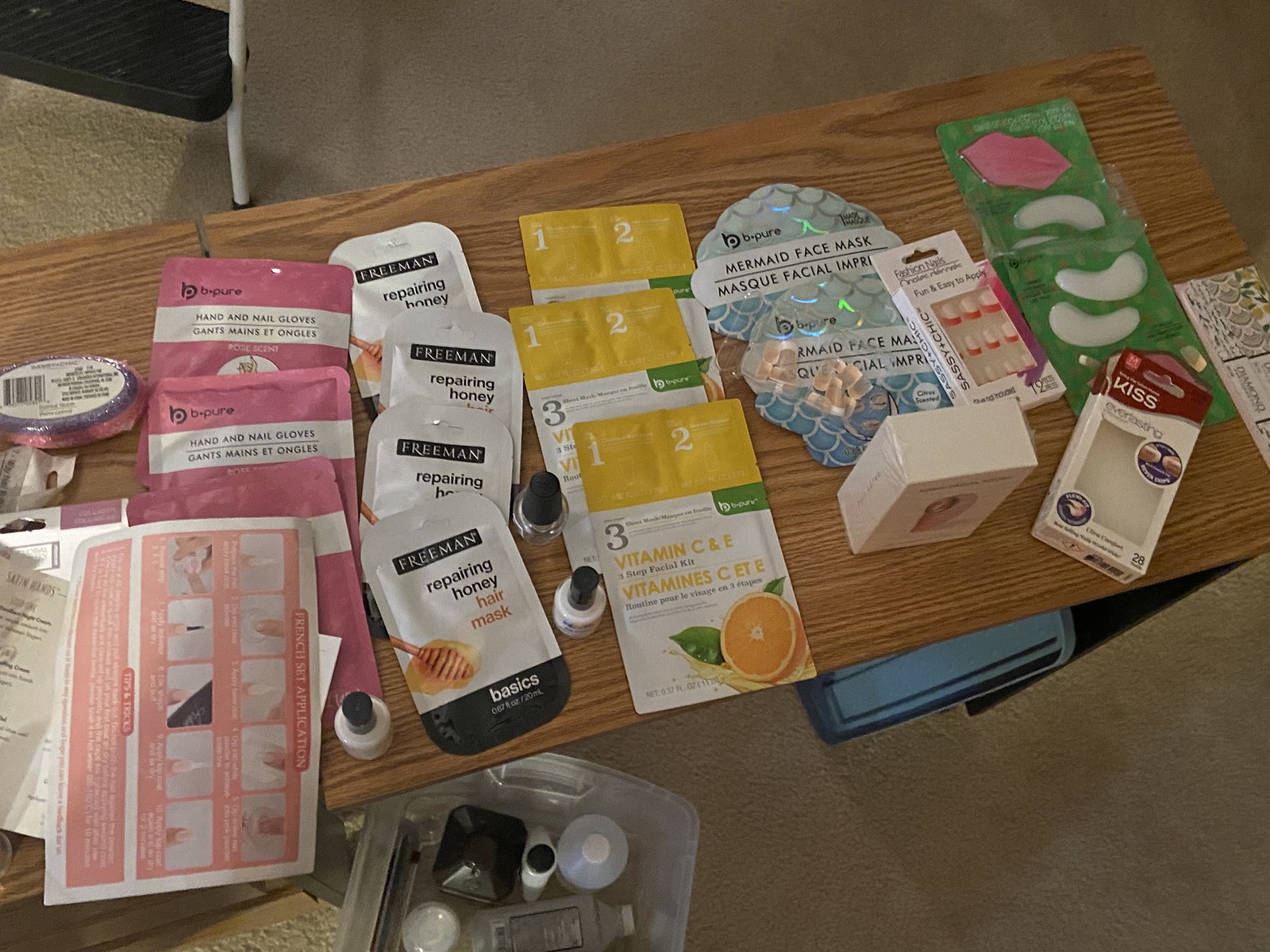This is a meticulously organized photograph showcasing an assortment of personal beauty and face products arranged neatly on an oak-colored laminate desk. The scene captures the attention with a series of carefully curated items:

On the left, a pink bar of soap with a white label trimmed in purple, detailed with black text and a UPC symbol, stands out atop a stack of instruction papers. These papers appear to provide guidelines for applying nail polish, featuring images of fingernails adorned with polish, in pink and white hues.

Adjacent to the soap, there are three packages of "Be Pure" hand and nail gloves, recognizable by their distinctive pink packaging and white stripe labeled in black text, accompanied by a corresponding French translation.

Next, a collection of four "Freeman" Repairing Honey Hair Masks sits in white packages, each decorated with a honey dispenser image. The packaging also features a black border with "Basics" inscribed in white at the bottom.

The arrangement continues with two bottles of nail polish - one clear, one white - flanking these hair masks, and another white bottle situated to the right.

Three additional packages emblazoned with "Vitamin C and E" imagery follow. These packages feature a yellow and white design highlighting an orange sliced in half, complete with green and white text.

Adding to the variety are two iridescent "Mermaid Face Masks" from "Be Pure," showcasing a color gradient from white to aqua, accented with a white band inscribed in black. A cellophane bag of pink press-on nails with white tips rests atop one of these masks.

In front of the face masks lies a white box presenting the back of a blonde woman's head, styled in a bun. Nearby, a package of "Fashion Nails" in pink with dark pink tips, branded as "Sassy and Chic," complements the collection. Additionally, there is an empty "Kiss" press-on nails box, identifiable by its maroon strip and clear cellophane front, showcasing images of the nails.

Completing the display, a green package contains under-eye pads in a curved shape and lip pads in an exaggerated lip shape, both visible through clear cellophane.

In the background, partially visible over the beige carpet, are elements of a step stool with a black plastic step and white metal frame. The floor space also reveals a tote containing a mix of bottles: a brown bottle, a white bottle with a black lid, a clear bottle with a white lid, and a clear bottle of alcohol lying on its side, adding to the scene's detailed composition.